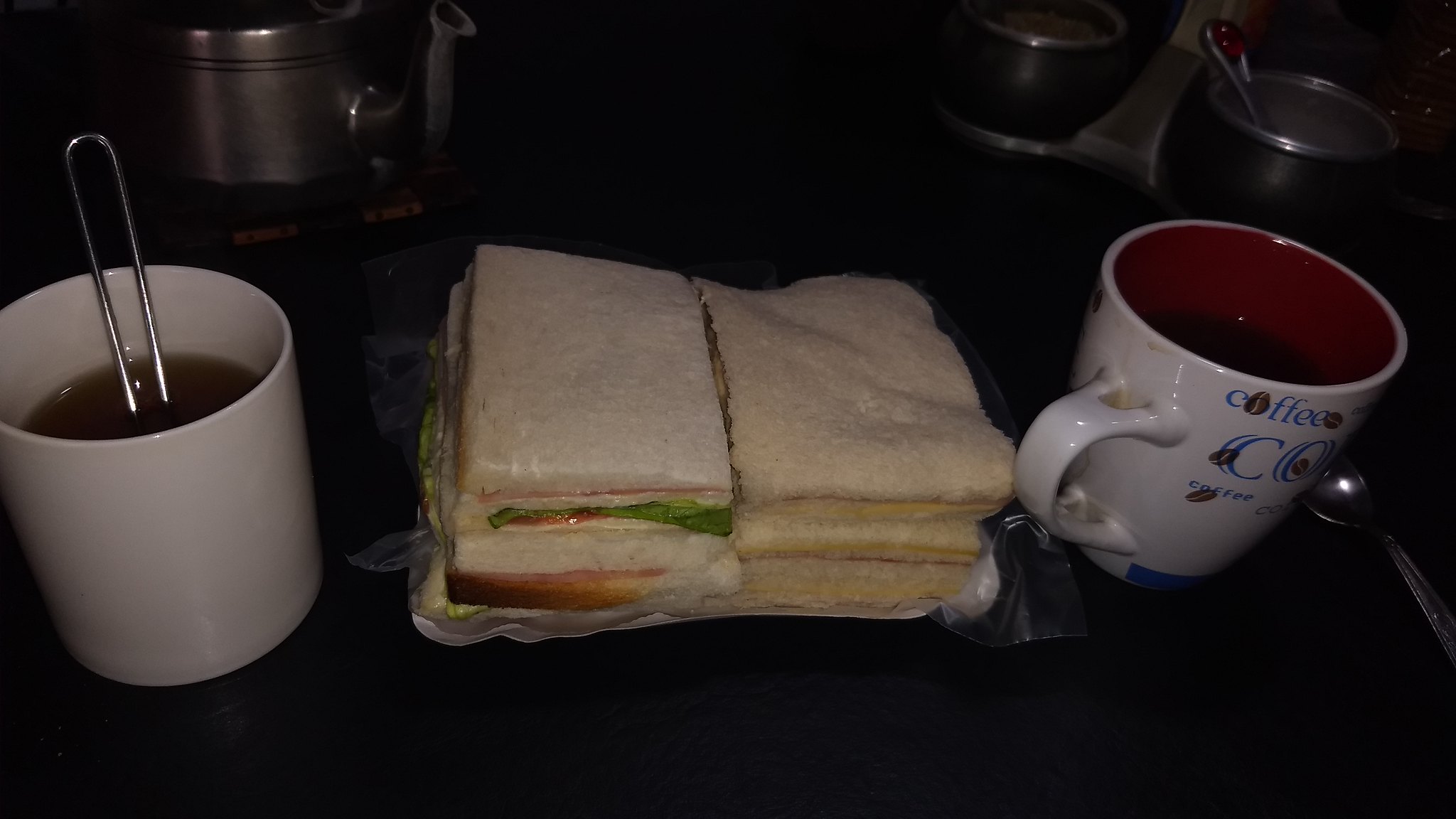In a dimly lit, indoor setting with a nearly black background obscuring finer details, this photo captures a tabletop scene featuring a spread of sandwiches and coffee mugs. Centrally positioned, there are two Dagwood-style sandwiches, expertly stacked and wrapped in plastic, made with crustless white bread. Visible ingredients include lettuce, cheese, ham, and possibly tomato. Surrounding the sandwiches are two ceramic mugs containing a dark liquid, likely black tea or coffee. The mug on the left is plain white with a silver utensil poking out, while the mug on the right is white with blue text that reads "coffee," featuring a red interior. In the background, there's a hint of metallic kitchenware, such as pots and pans, adding subtle reflective highlights to the otherwise dark composition.